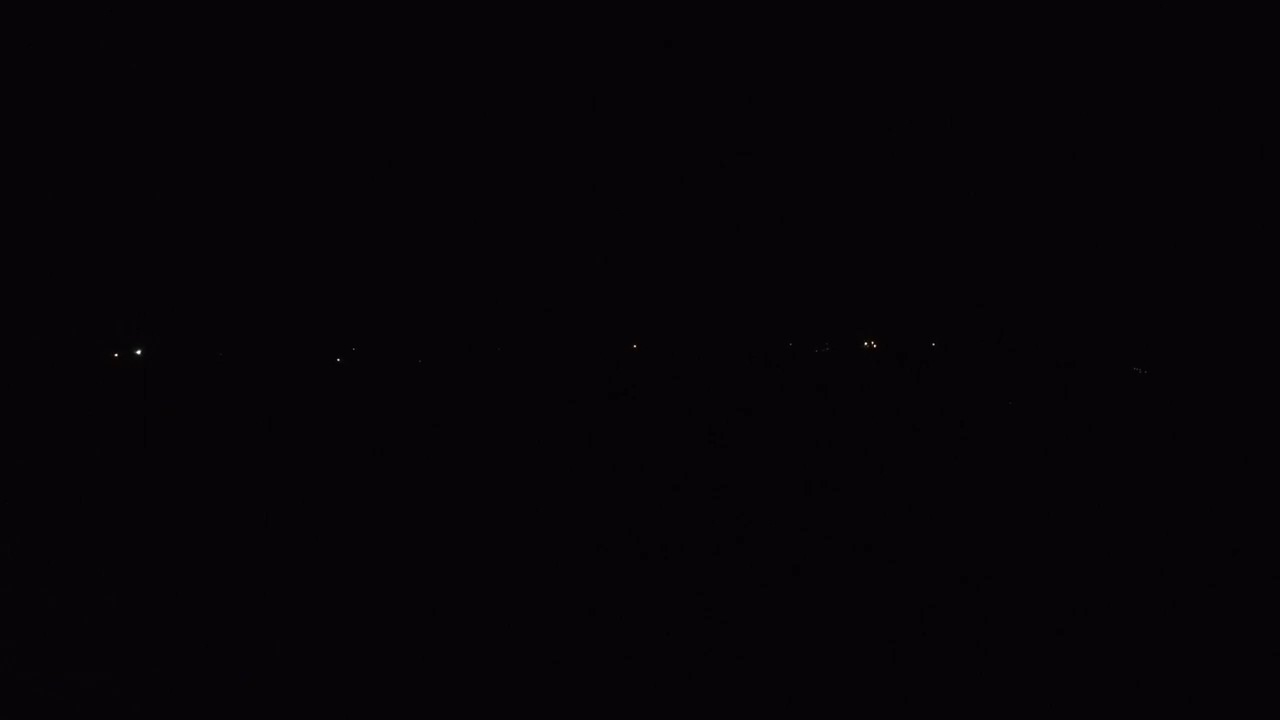The image appears predominantly black, with over 99% of it shrouded in darkness, resembling a black square or rectangle. In the middle, there is a horizontal array of tiny light spots that break the vast blackness. There are around seven or eight small white dots, uneven and inconsistent in size and spacing. From left to right, the sequence includes a small dot followed by a larger one, a gap, another dot with a tiny one next to it, another gap, a single dot, and then a cluster of three dots before one final white spot. These dots are the only elements disrupting the otherwise blank blackness of the image.